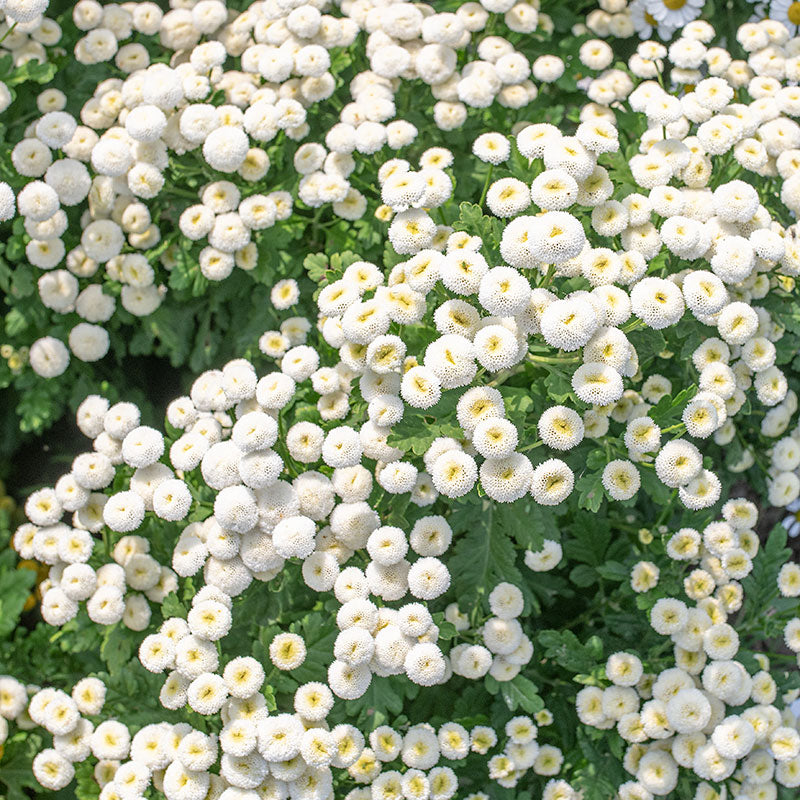This photograph captures a dense and lush scene of flowering plants, prominently featuring hundreds of circular white flowers with yellow centers. The flowers, abundant and thick, dominate the image from top to bottom, creating a vibrant and lively display. The petals form intricate patterns, almost resembling tiny dots or scallops, and the rich, multi-dimensional layers of flora contribute to a captivating depth. Behind the white blooms, the backdrop is filled with a lush combination of lime and deep green leaves. Bathed in a soft, morning light that imparts a gentle glow, the picture exudes tranquility and hints at a warm, summery climate. The absence of any text allows the natural beauty of the green, white, and yellow hues to speak for themselves, making it a visually engaging and serene scene.